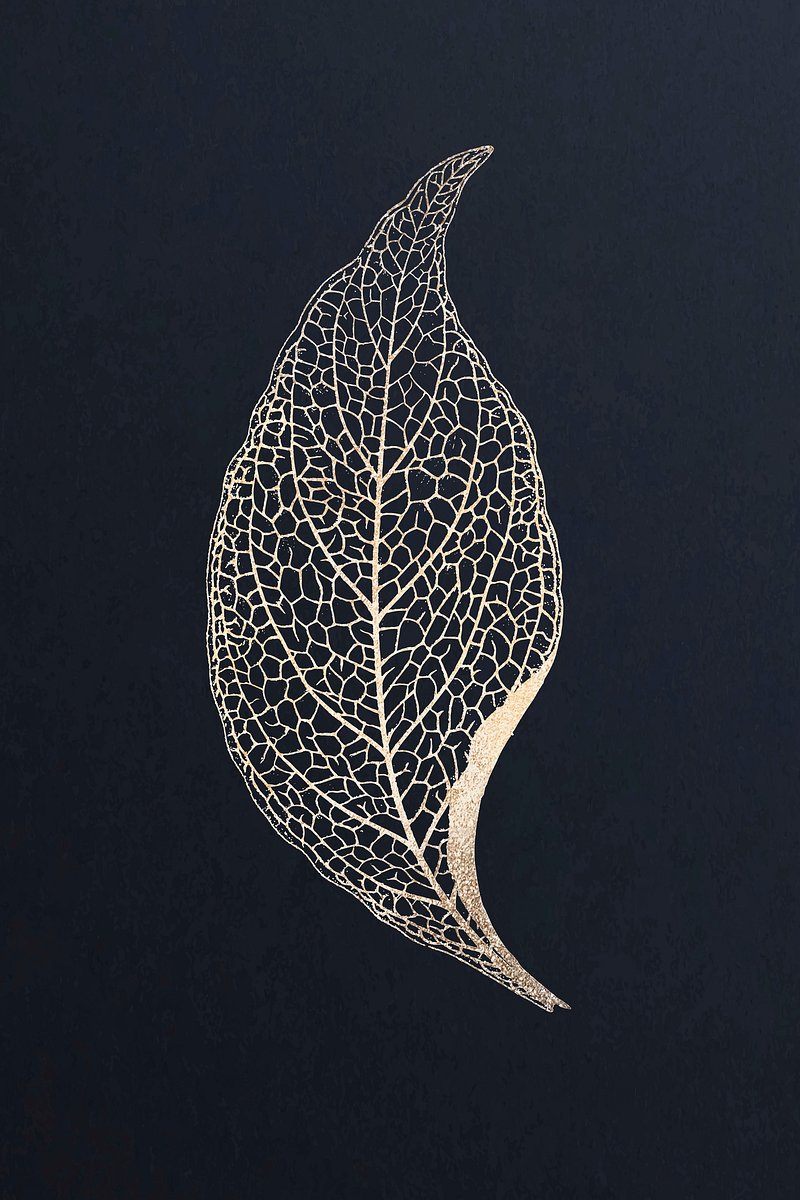In this rectangular image, approximately 6 inches high by 3 inches wide, a single gold leaf is the focus. Set against a black backdrop that could be either fabric or paper, the leaf is about 3 inches high, with its widest point stretching 1.5 inches across its center. The leaf's design starts towards the bottom right corner, curving gracefully to the left before arching back up to the right, forming a familiar and natural leaf shape. The leaf has a shiny, glittery appearance, achieved with gold glitter paint. At its center, a thin main vein branches out diagonally into smaller veins, giving the leaf intricate, detailed structure. The black background peeks through these veins, creating a striking contrast. The overall depiction is more artistic than realistic, featuring thin and thick lines that produce a somewhat translucent effect in places. The leaf's decorative sparkle, particularly prominent on the right side, adds to its vivid, ornate presentation.